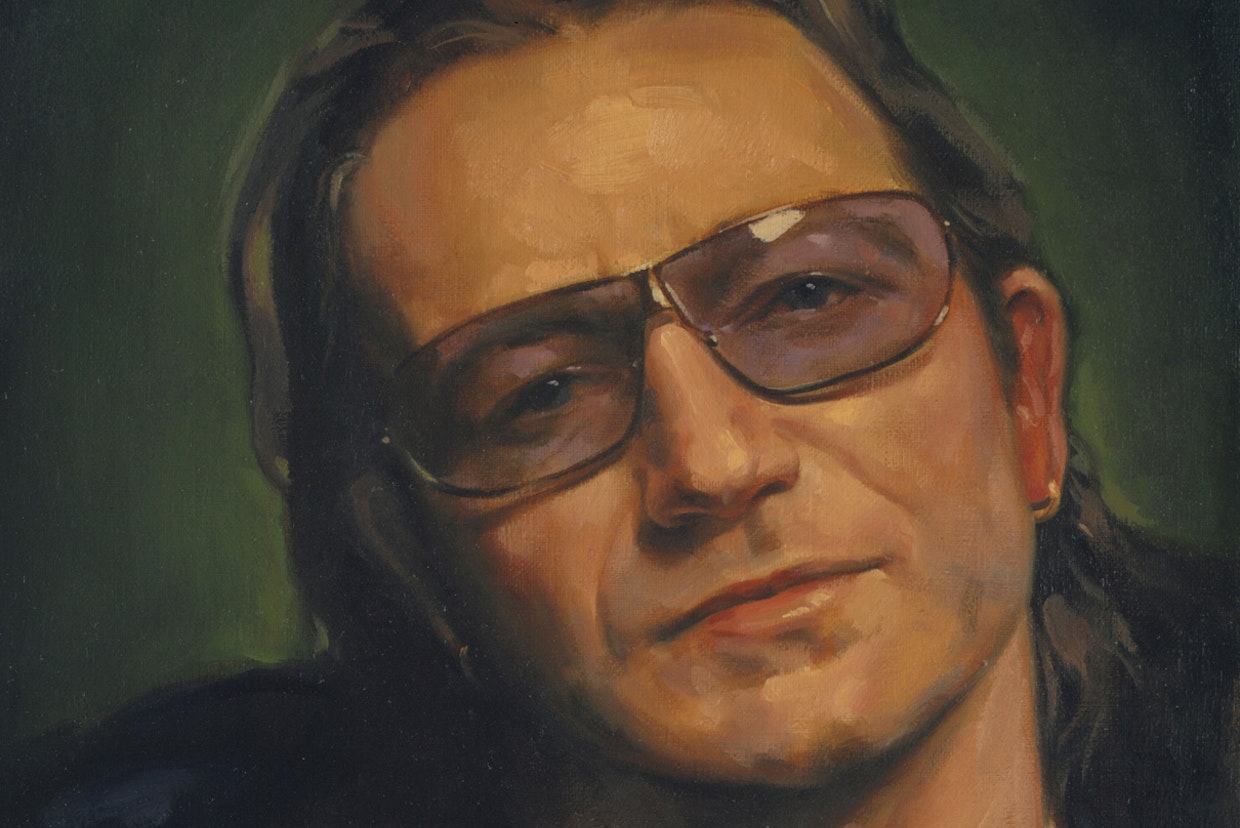This painting depicts the face of Bono, the lead singer of U2. His head is slightly tilted to the left, and he is gazing directly at the viewer. Bono's complexion shows a mix of brown and blue tones, adding depth to his face. He is wearing gold-rimmed sunglasses with a slight purple tint that partially obscure his blue eyes. His long, dark brown hair, which is tucked behind his ears, ends just at the top edge of the painting. Small gold hoop earrings are visible on both ears. Bono is dressed in a dark shirt or jacket, possibly black, as can be glimpsed at the top of his shoulders. The background features a gradient that starts with a light green glow around his face and transitions to a darker green towards the edges, creating a spotlight effect that emphasizes his presence. The left side of his face is shaded, with more light illuminating the right side, giving a three-dimensional quality to his visage.